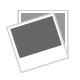This photograph features a metallic flashlight that is prominently displayed against a flat white surface. The flashlight, likely made of aluminum, exudes a utilitarian and minimalist aesthetic, designed with function in mind rather than ornamentation. The entire exterior, from the grip to the beam, is crafted from shiny, reflective metal, indicating it's possibly taken outdoors as evidenced by a strong, bright reflection. 

Positioned with its light-emitting end in the lower right corner, the flashlight reveals a very small bulb encased within a clear, reflective enclosure. Although not illuminated, the bulb is easily visible through the clear lens. The handle of the flashlight is medium length and includes numerous small indentations, presumably to enhance grip. These indentations are accompanied by lines engraved into the metal, which may have accumulated some dirt, creating the appearance of black stripes. The overall appearance suggests a durable, practical device, perhaps even slightly weathered from use.

A subtle characteristic of the background includes a faint fold towards the top, indicating the possibility of a backdrop, which supports the notion that this could be a professional photograph intended for advertising. The flashlight also features a cap at the end of the handle, likely for battery placement.

In summary, the image captures a thick, silver, metal flashlight with a clear emphasis on its reflective properties and functional design, set against a white, slightly textured background.